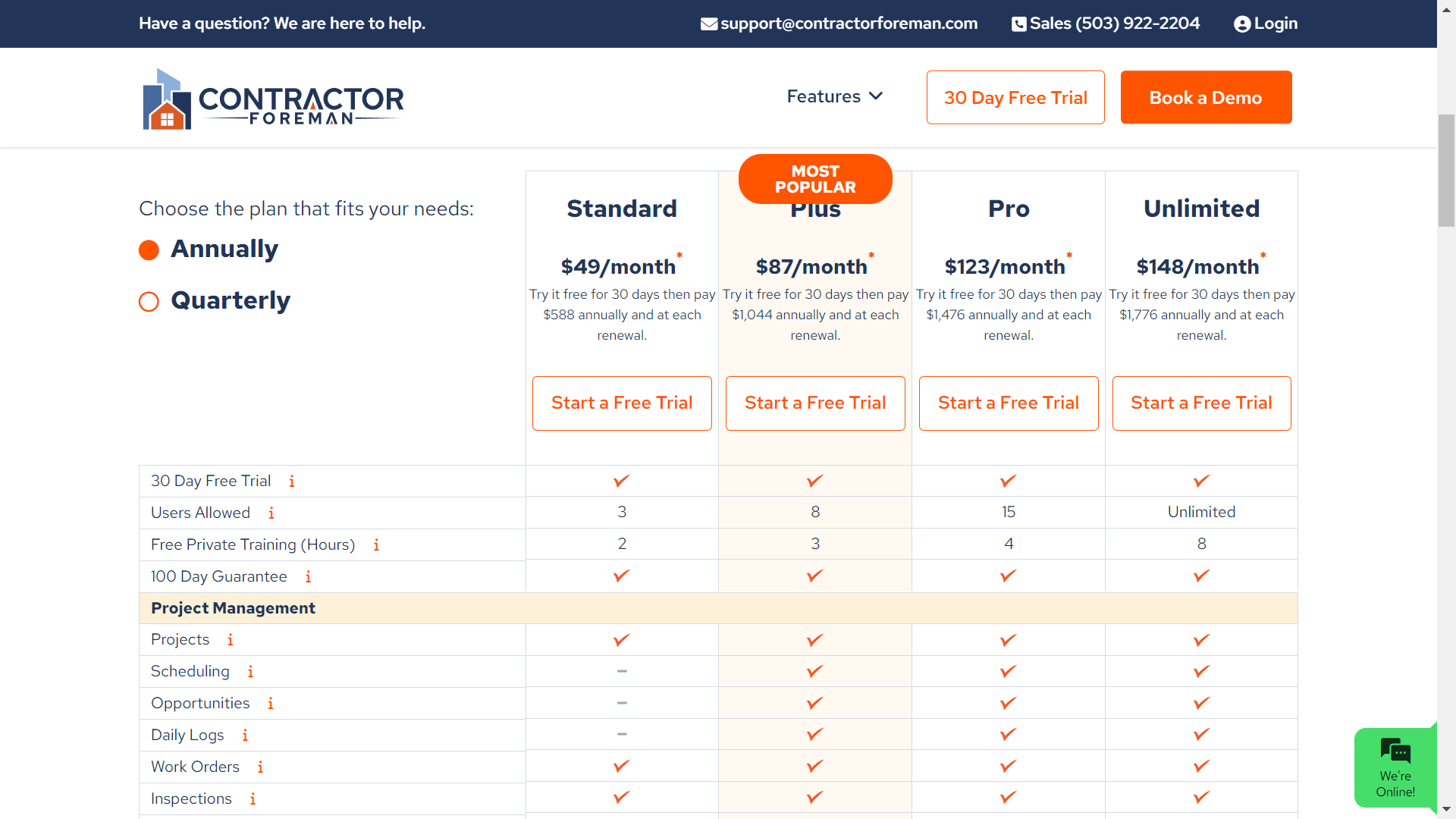Located at the top of the image, there's a long blue bar that reads, "Have a question? We are here to help," with a "Log In" option adjacent to it. Below this, the text "Contractor Foreman" is displayed alongside a red image of a house set against a blue background. To the right, an arrow pointing downward indicates additional options. Further down, an orange-outlined square promotes a "30 Day Free Trial," with a solid orange square offering the option to "Book a Demo."

Beneath this section, the heading "Choose the plan that fits your needs" is prominently displayed. Next to it, an orange circle labeled "Annually" and a white, orange-outlined circle labeled "Quarterly" are positioned side-by-side. To the far right, an orange-circled label reads "Most Popular." The pricing plans are listed as follows: the "Standard" plan at $49 per month, which is not specially highlighted; the "Plus" plan at $87 per month, also marked "Most Popular" and outlined in orange; the "Pro" plan at $123 per month; and the "Unlimited" plan at $148 per month. Each plan has a "Start a Free Trial" button underneath.

On the left side of the pricing options, a variety of features are listed, with "Project Management" specifically highlighted in a light orange rectangle. Finally, in the bottom right corner, a green box states, "We're Online."